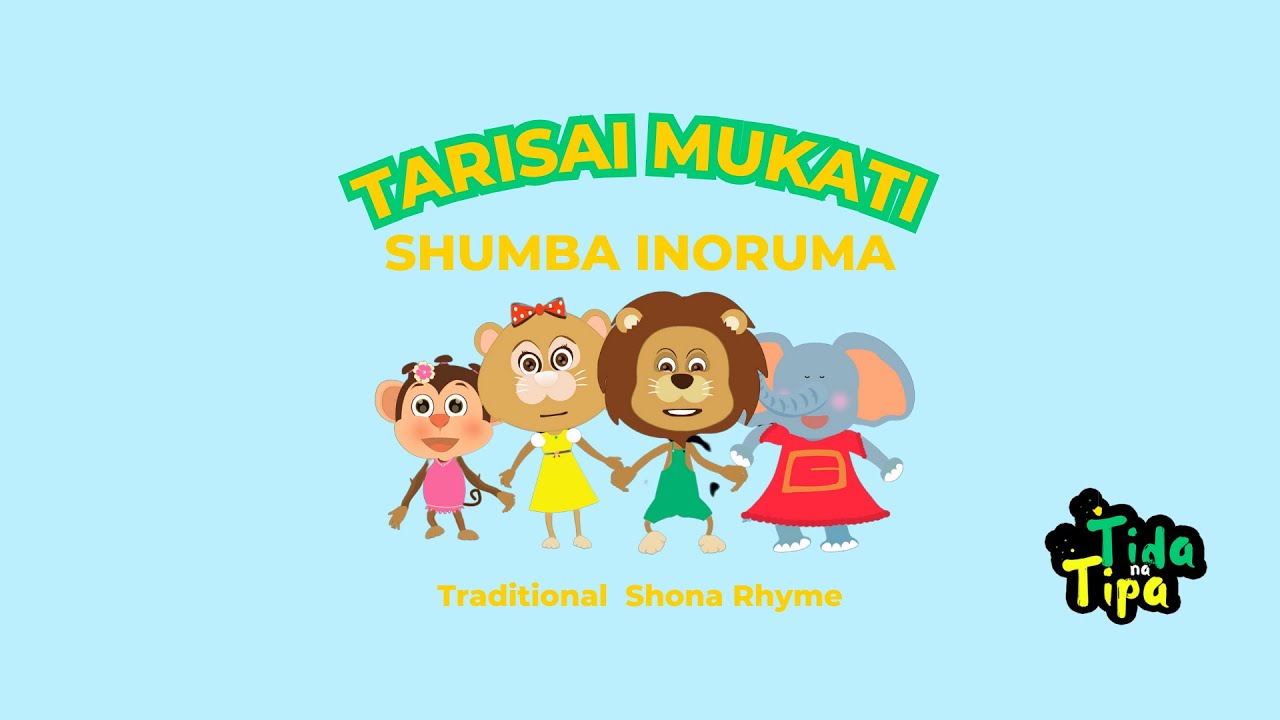The rectangular image, wider than it is tall, features a baby blue background with vibrant visual elements. In the bottom right corner, a small design displays "Tida Tipa Na Tipa." At the center, four cartoon characters—an elephant, a lion, a mouse, and a monkey—stand in a row, holding hands and dressed in bright colors. The elephant wears a red dress, the lion is in green overalls, the mouse sports a yellow dress, and the monkey dons a pink dress. All but the monkey are wearing white shoes. Above the characters, in yellow block letters with a green border, the text reads "Terasai Mukati" followed by "Shumba Inoruma" and, below that, "traditional Shona rhyme." The image appears to advertise a children's show or book featuring a traditional Shona rhyme.